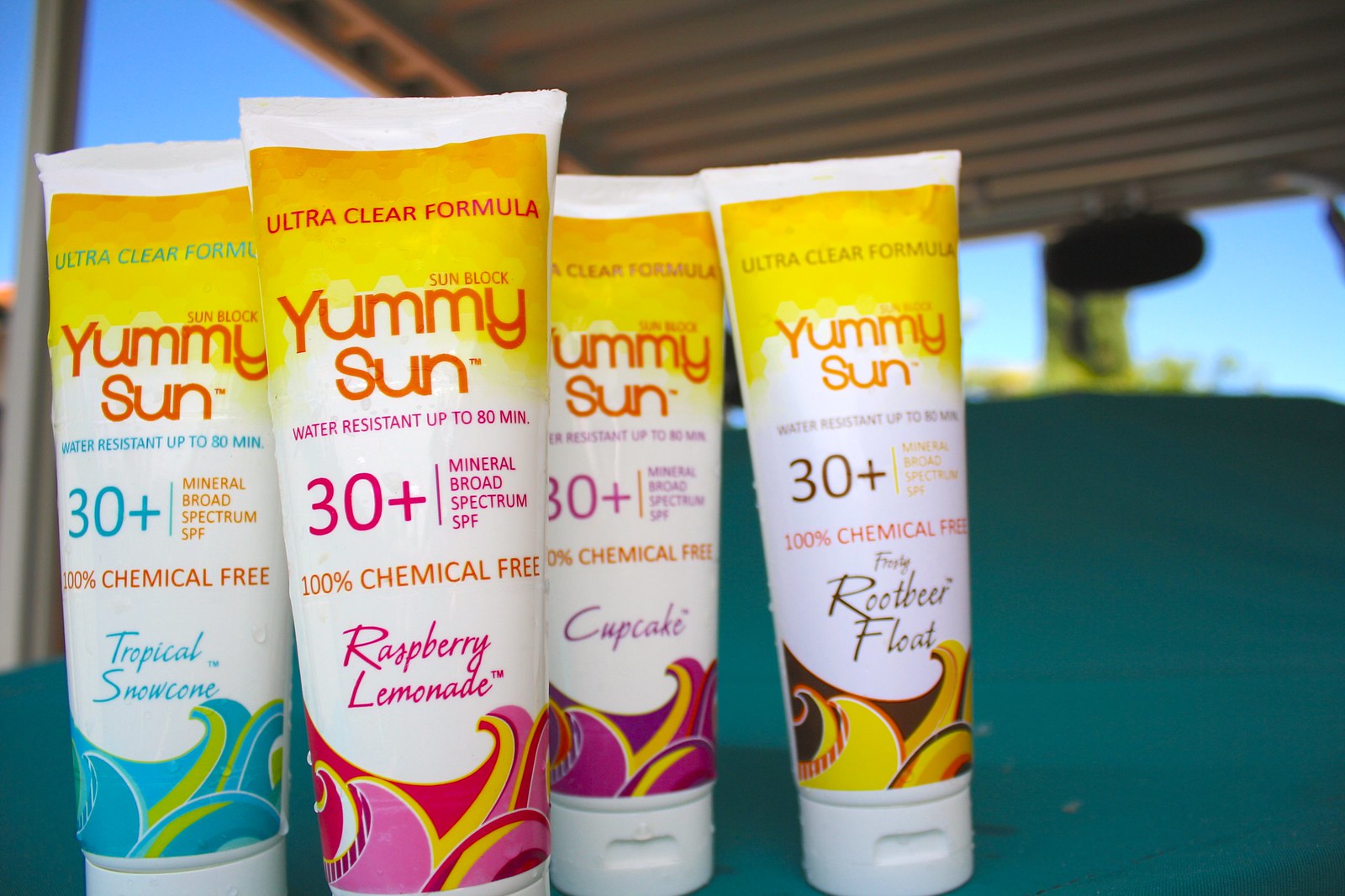The photograph features four colorful tubes of suntan lotion by the brand Yummy Sun, lined up on a green table outside. Against a backdrop of a blurred blue sky, a roof with visible indentations, a supporting pole, and a black unidentified object, the vivid colors of the suntan lotions stand out prominently. Each tube, positioned upside down with the openings facing downward, is highlighted by a striking yellow band across the top displaying the text "Ultra Clear Formula."

Every tube boasts 30+ SPF protection and is labeled as "100% chemical-free, mineral broad-spectrum SPF." Each lotion has a unique scent, indicated by vibrant colors and themed waves near the base of the tubes. The tube on the far left, "Tropical Snow Cone," features a blue and white design with a blue wave. Next is the "Raspberry Lemonade" tube in pink with a red wave. The third tube, marked "Cupcake," carries a magenta color scheme with a dark purple wave. Finally, the far-right tube, labeled "Root Beer Float," displays a brown and yellow design with a corresponding wave at its base.

All four tubes enhance the sunny outdoor setting with their cheerful and varied appearances, reflecting the playful essence of Yummy Sun's product line.